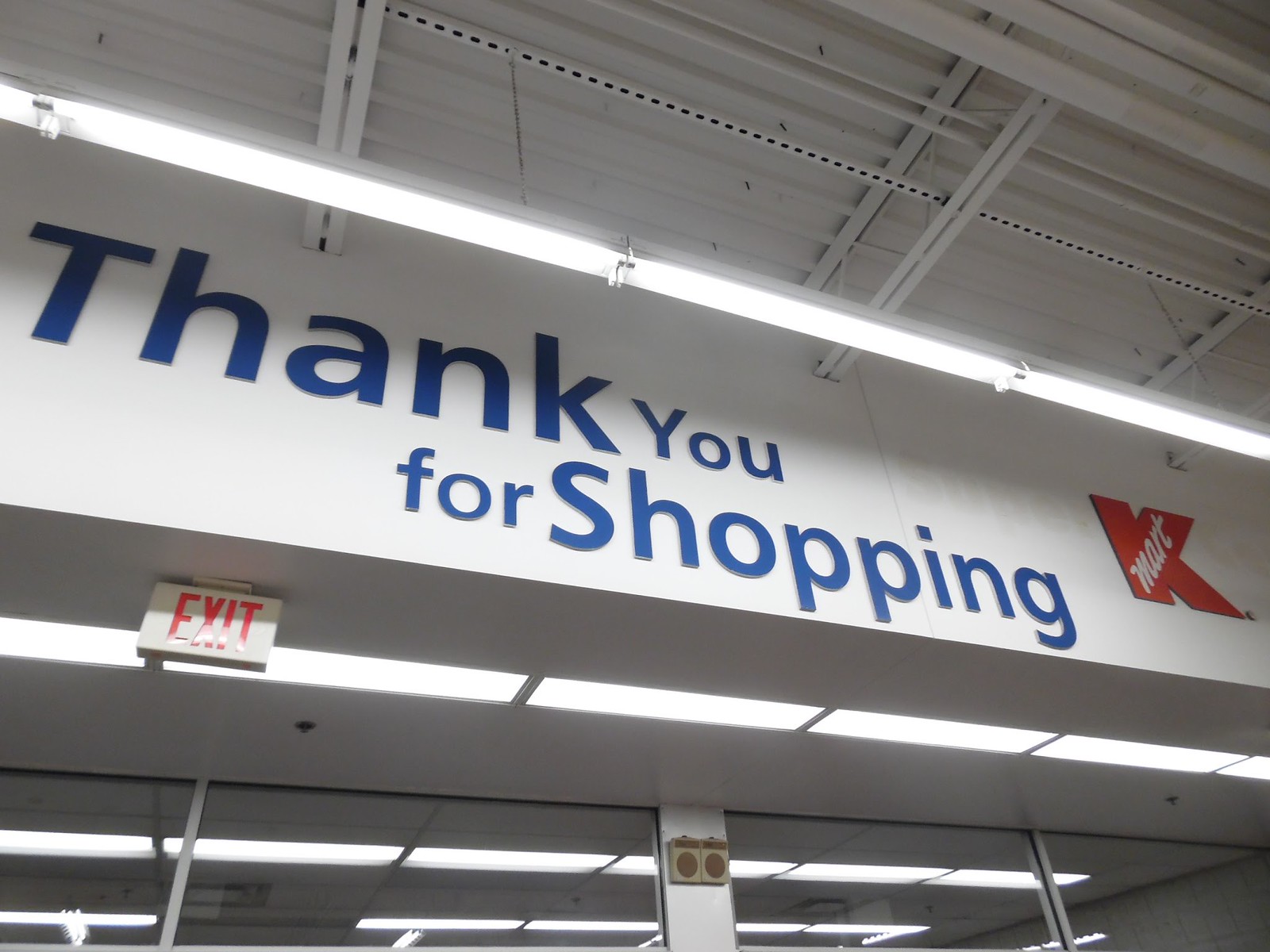This photograph captures the overhead view at the entrance of a Kmart store, just as if you were about to exit. Prominently displayed high on the wall is a large blue "Thank you for shopping" sign with "thank" and "shopping" in a larger font size. To the right of the text is the iconic red Kmart logo, featuring a red "K" with "mart" written in white cursive letters. The industrial ceiling, lined with strips of white metal and a long linear fluorescent light fixture, frames the scene above. Below the sign, the familiar red rectangular exit sign hangs, with the tops of glass doors and windows visible beneath. The wall also features a metal post which may be part of an alarm system, adding to the practical, utilitarian feel of the store's design.